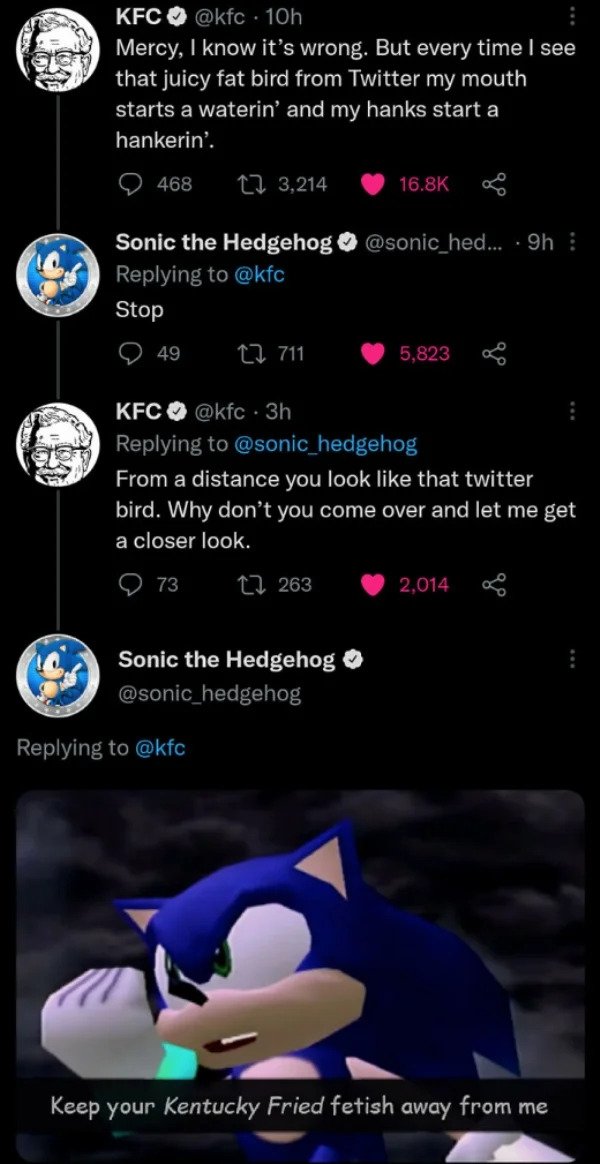Here's a cleaned-up and descriptive caption for the image:

---

**A Humorous Twitter Exchange Between KFC and Sonic the Hedgehog**

In this image, a Twitter conversation unfolds between the verified accounts of KFC and Sonic the Hedgehog. KFC’s account is represented by the iconic black and white drawing of Colonel Sanders, while Sonic the Hedgehog’s account is marked by an illustration of the blue and brown hedgehog.

On a black background, at the top, we see a tweet from KFC (@KFC) posted 10 hours ago. KFC humorously tweets, "Messi, I know it's wrong, but every time I see that juicy fat bird from Twitter, my mouth starts watering and my hands start hankering." This tweet has garnered significant engagement, including 468 comments, 3,214 retweets, and 16.8k likes.

Sonic the Hedgehog (@SonicTheHedgehog) replies sharply, "Stop." This reply also marks 10 hours ago, indicating a prompt response.

KFC then cheekily responds, "From a distance, you look like that Twitter bird, why don't you come over and let me get a closer look."

In a final rebuttal, Sonic the Hedgehog retorts, "Keep your culinary fetish away from me," raising his fist and facing towards the left, signifying his defiance towards KFC's quirky advances.

This playful banter between KFC and Sonic the Hedgehog adds a humorous touch to the otherwise mundane platform, highlighting the engaging personalities of brand accounts on social media.